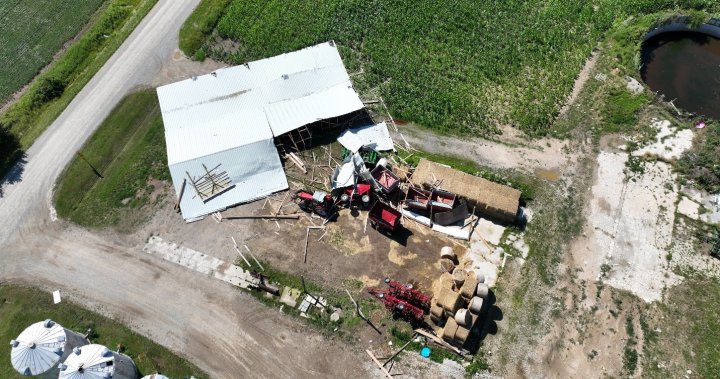This aerial photograph captures the aftermath of severe weather damage, likely caused by a tornado or a heavy storm, in a rural area dominated by grassy fields and trees. In the bottom left of the image, there are prominent grain silos. A dirt road leads directly up to the epicenter of the devastation, where a large shed-like building with a white roof has suffered significant damage, evidenced by the roof being completely blown off and scattered debris, including lumber and various farm vehicles such as tractors and wheelbarrows, strewn about. Adjacent to the damaged white-roofed building is a long structure with a brown roof that remains intact. The overall scene is one of destruction, with scattered sticks and wreckage indicating the force of the weather event. Despite the widespread damage, no human beings are visible in the image.